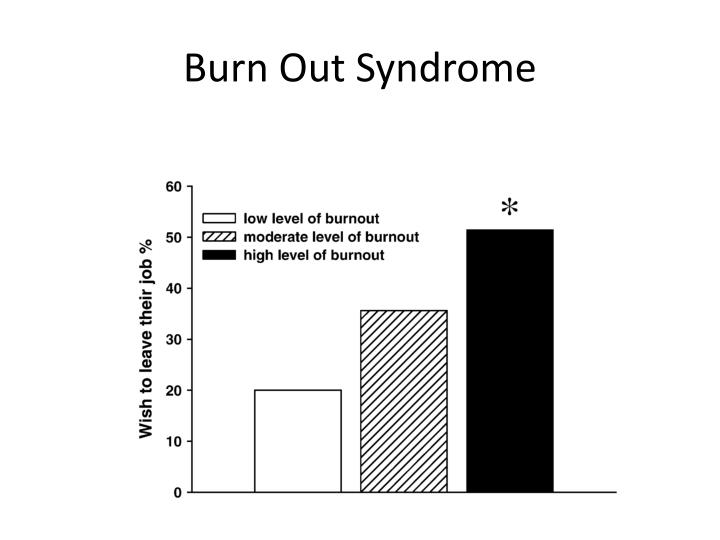The image features a bar graph against a white background, devoid of a border. The title in bold black letters at the top reads "Burnout Syndrome." Along the left vertical axis, labeled "Wish to Leave Their Job Percentage," the scale ranges from 0% to 60%. The graph comprises three bars indicating different burnout levels among employees. The first bar, filled in white, represents a low level of burnout at 20%. The second bar, marked with diagonal black stripes, denotes a moderate level of burnout at approximately 35-40%. The third bar, completely black and distinguished by an asterisk above it, signifies a high level of burnout at 50%. Additionally, horizontal and vertical black lines guide the viewer through the percentage levels for clarity.